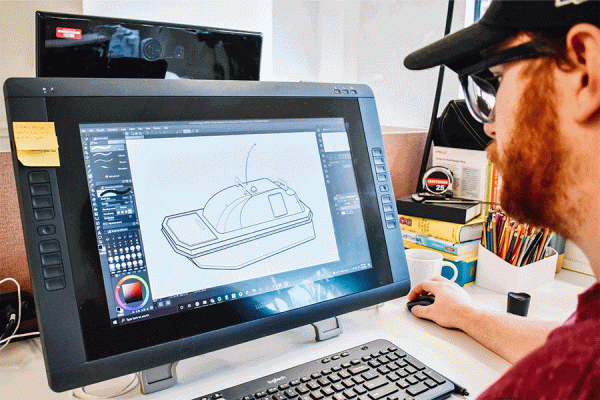In the image, a man is seated at a desk, engrossed in graphic design work on his computer. He is modeling a 3D CAD depiction that appears to be a sleek, white boat with a balloon-like border. The man, who has a striking orange or reddish beard, is wearing a black baseball cap and black-framed glasses. He is also dressed in a dark red shirt. The scene captures his side profile, with one arm positioned on the mouse as he intently stares at the illuminated computer screen. The workspace includes a black keyboard, with a noticeable shine reflecting off the screen, and a second monitor behind the main one. Additional details in the background include a white box of colored pencils and some books, emphasizing the creative nature of his work environment.